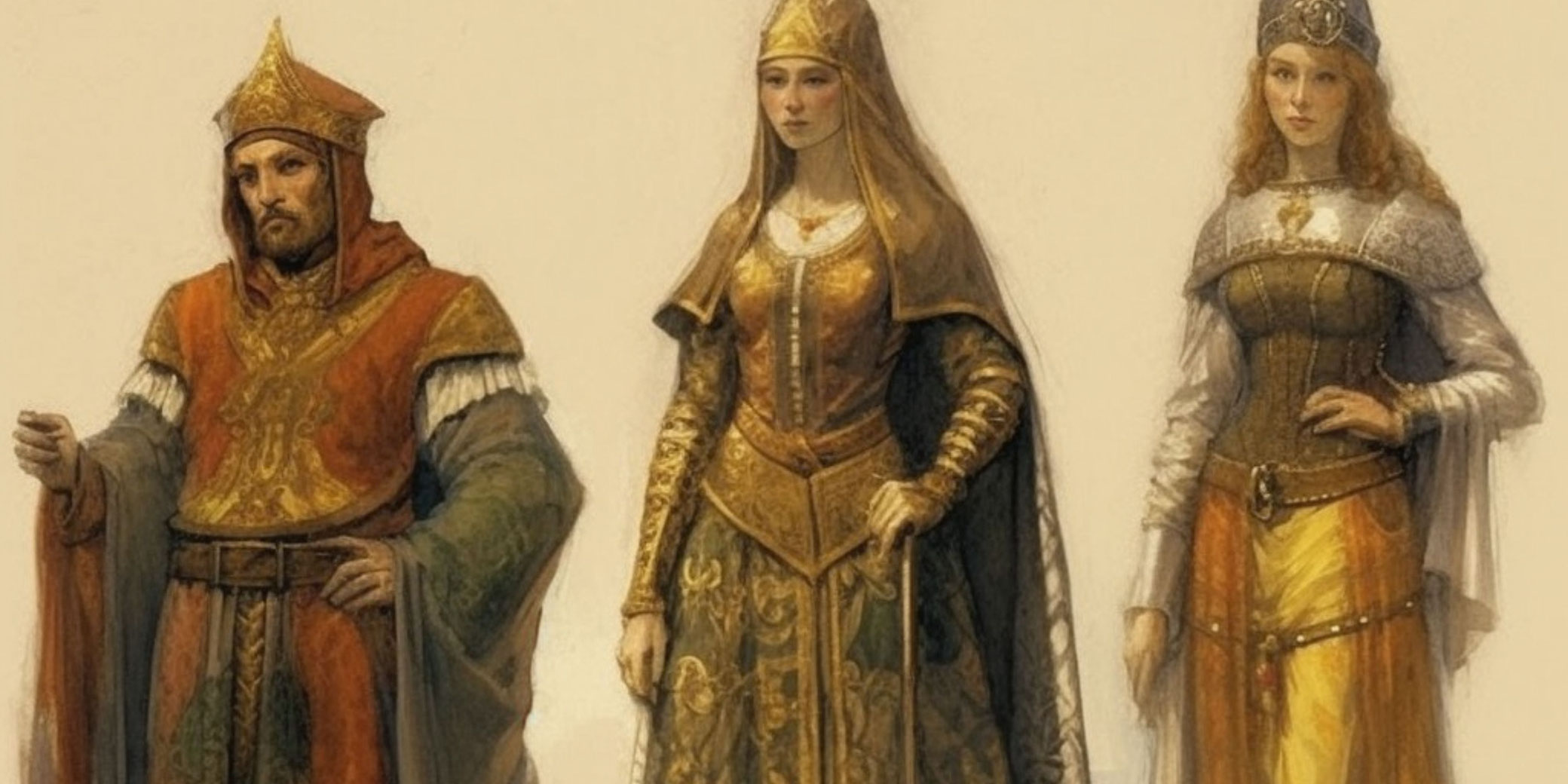This is a historical-style illustration portraying three figures from medieval times, likely from a European context such as Spanish, Portuguese, or Italian. The Catholic Church's influence is evident in the attire and composition. 

On the left stands a man dressed in a long, medieval robe predominantly in shades of red and orange, with a gray and gold center and a brown belt. His head is covered by a pointed hat that includes a hood, featuring a gold top and red backdrop. He holds one fist up in the air while his other hand rests on his waist.

Beside him, the first woman is adorned in an elegant, golden two-piece dress, her pale skin accentuated by red rouge on her face. Her golden headdress covers most of her forehead and drapes into a cloak over her shoulders. She holds a staff in one hand, and the dress flows into a flowery design at the bottom.

The second woman stands next to her, showcasing curly red hair under a blueish or metallic crown. She wears a three-piece suit that includes a green shirt with gray sleeves, a corset, and a skirt in shades of silver, gold, brown, and orange. A piece of porcelain-like armor covers her shoulders, and her left arm is assertively placed on her hip.